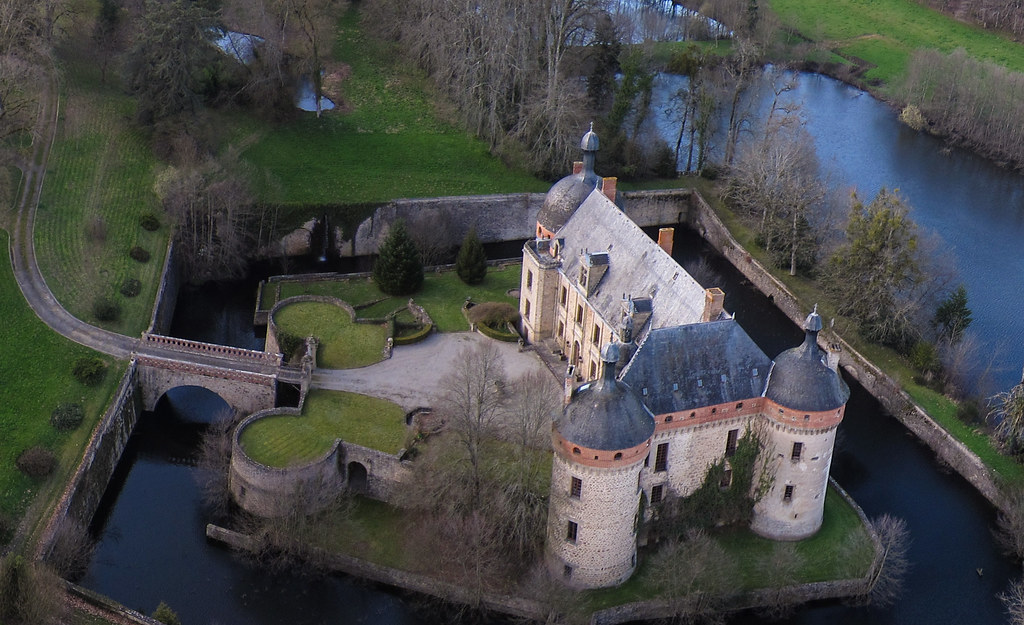The image captures an outdoor scene taken during the day, showcasing a grand, multi-level building positioned slightly to the right of the center. The structure appears to be constructed from bricks or stone, though the distance makes it difficult to specify. The base of the building exhibits a grayish facade, while its roofs display a combination of dark bluish-black and orange hues. Above this section, the main portion of the house features light brownish walls with a grayish roof. Further up, another segment of the building replicates the design of the initial portion, with a black roof and orange detailing.

To the left of the building, a long, grayish roadway stretches towards the entrance. Surrounding the house is a lush, green grassy area that adds a vibrant contrast to the scene. Additionally, the building appears to be encircled by water, forming a moat-like feature. On the far right, a substantial body of water, resembling a pond, displays a dark blue or almost black coloration.

In the background, the top middle section of the image is adorned with numerous tall, old trees, featuring brown trunks and reaching high into the sky. These elements contribute to the picturesque and serene atmosphere of the photograph.